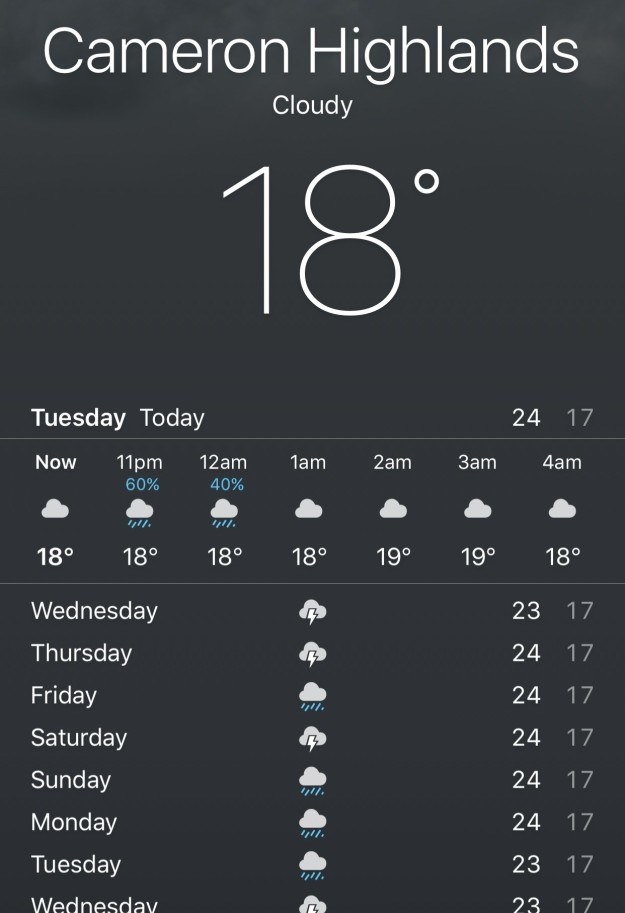The image is a screenshot resembling a phone display, showcasing a comprehensive weather forecast for the Cameron Highlands. The entire background is black, with white text providing the details, and light blue text highlighting a strong chance of rain.

At the top, "Cameron Highlands" is prominently displayed in large white letters. Beneath it, in slightly smaller text, it reads "Cloudy." Dominating the center, the current temperature is shown in gigantic digits: "18°C."

Directly below, it notes "Tuesday" and "Today," with a high of 24°C and a low of 17°C for the day. The forecast provides hourly updates: at "Now," it shows cloudy skies and 18°C. For 11:00 AM, there is a 60% chance of rain, still at 18°C; at 12:00 PM, the chance of rain drops to 40%, remaining at 18°C, followed by hourly temperature predictions of either 18°C or 19°C through to 4:00 AM.

The extended outlook begins with "Wednesday" and displays a mix of clouds and chances of rain consistently throughout each day of the week. Specifically, Wednesday shows temperatures ranging from a high of 23°C to a low of 17°C. The pattern remains largely unchanged with Thursday, Friday, and the following Monday, all forecasting highs of 24°C and lows of 17°C. The next Tuesday and Wednesday predict slightly lower highs of 23°C with lows of 17°C.

This detailed weather forecast provides both daily and hourly insights, ensuring residents and visitors of Cameron Highlands are well-informed of the upcoming weather conditions.